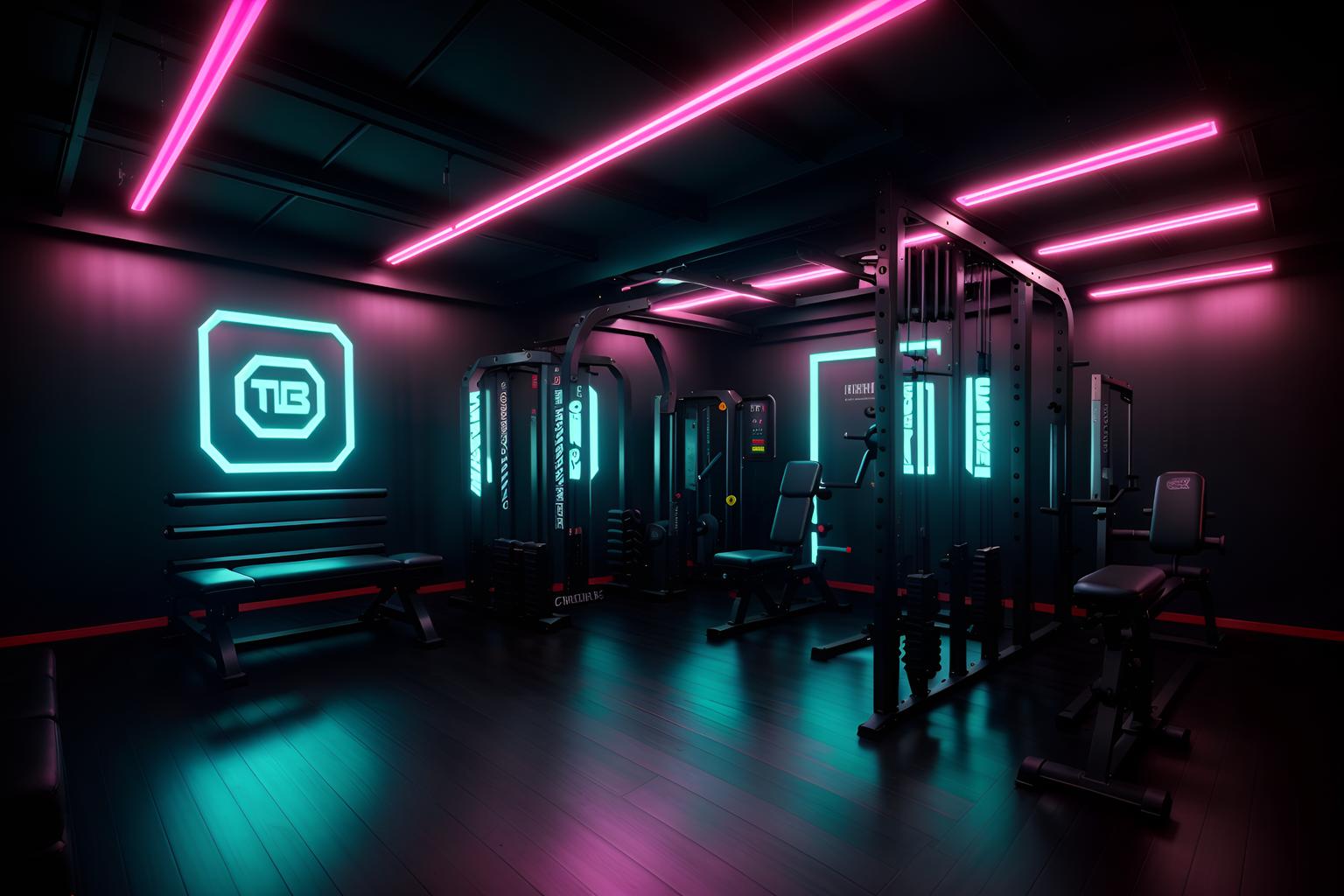The image depicts an advanced and expensive gym bathed in vibrant neon lighting against a very dark backdrop. The overall ambiance is dim, punctuated by bright blue and pink fluorescent lights. The ceiling is adorned with five long pink fluorescent light strips that create striking lines of light, while various blue fluorescent lights outline the walls. The gym features a dark brown to black hardwood floor that subtly reflects the colorful illumination. Centered is a weight bench situated beneath a distinctive square light fixture. This fixture comprises a square with rounded corners, within which resides an octagon bearing the initials "TB". The room appears furnished with sleek, black weight equipment, suggesting a modern, high-end aesthetic. Overall, the space exudes an exclusive, futuristic vibe.